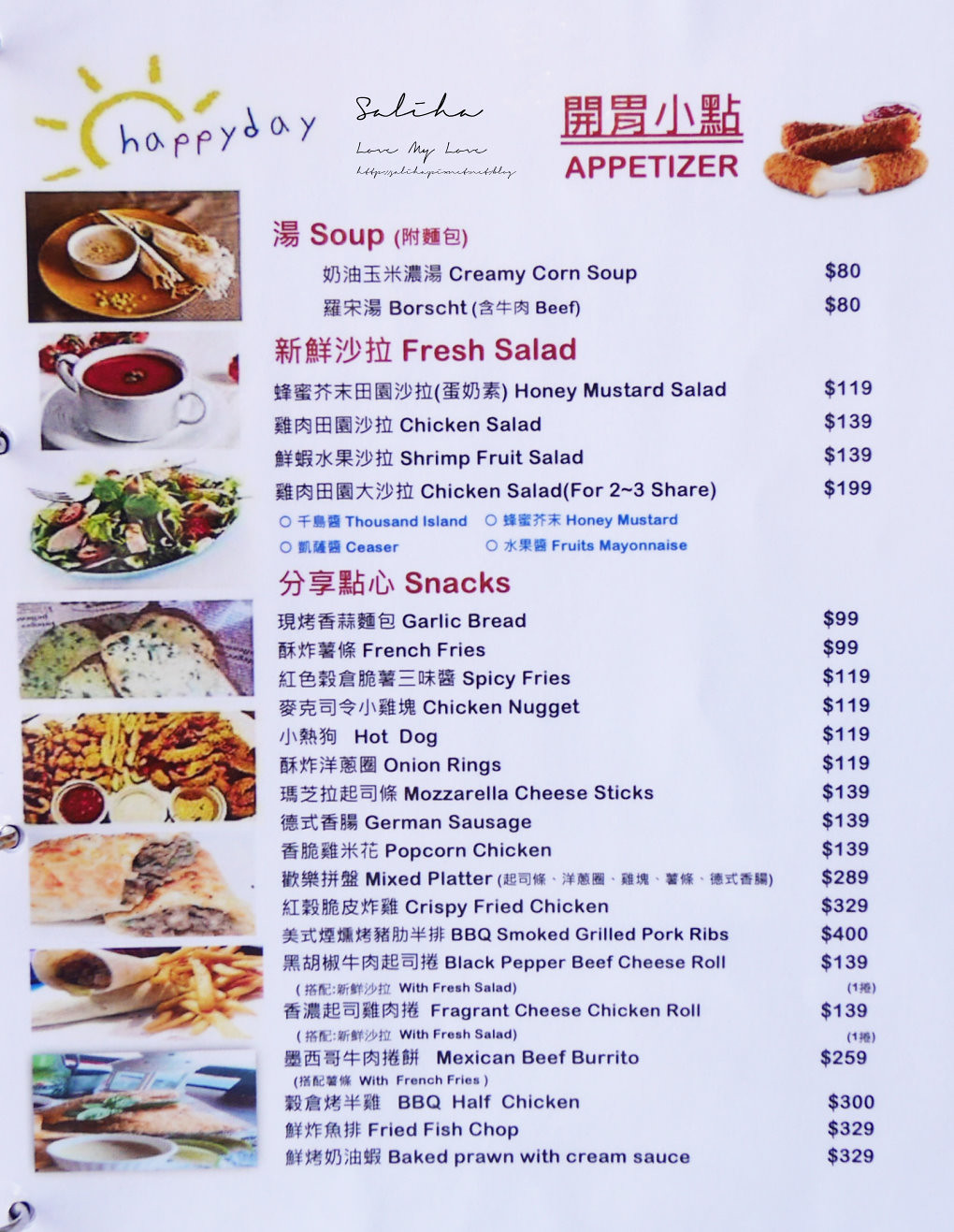The image features a vertically rectangular menu with a light background, which appears to be either white or very light gray. At the top of the menu, the phrase "happy day" is written in lowercase blue letters, accompanied by a yellow graphic of a half-risen sun, implying a cheerful and welcoming theme. 

Beneath the "happy day" text, there is some Asian writing, which is followed by the word "Salicha," though its meaning is unclear. Below this section, the menu lists items categorized by type, each prefaced with similar Asian writing, suggesting that the establishment might cater to an international clientele or is located in an Asian country.

The first section of the menu is titled "Appetizer" in red, with a realistic image of cheese sticks positioned at the top right of this section. Following this, the "Soup" category is indicated in red, listing various options in blue text:
- Creamy Corn Soup
- Borscht

Next is the "Fresh Salad" section, also in red, with the following items in blue:
- Honey Mustard Salad
- Chicken Salad
- Shrimp Fruit Salad
- Chicken Salad for 2-3 (to share)

Another section titled "Snacks" in red follows, listing several items in blue text. Adjacent to each listed item, there are prices displayed in what appears to be a non-US currency, such as 80, 119, and 139 units, respectively.

Additionally, realistic images of various food items such as soups, salads, chicken dishes, french fries, and tortillas are displayed along the left side of the menu, providing a visually appealing preview of the dishes offered.

The detailed menu layout, combined with clear images and multilingual text, suggests a diverse dining experience catering to different tastes and preferences.